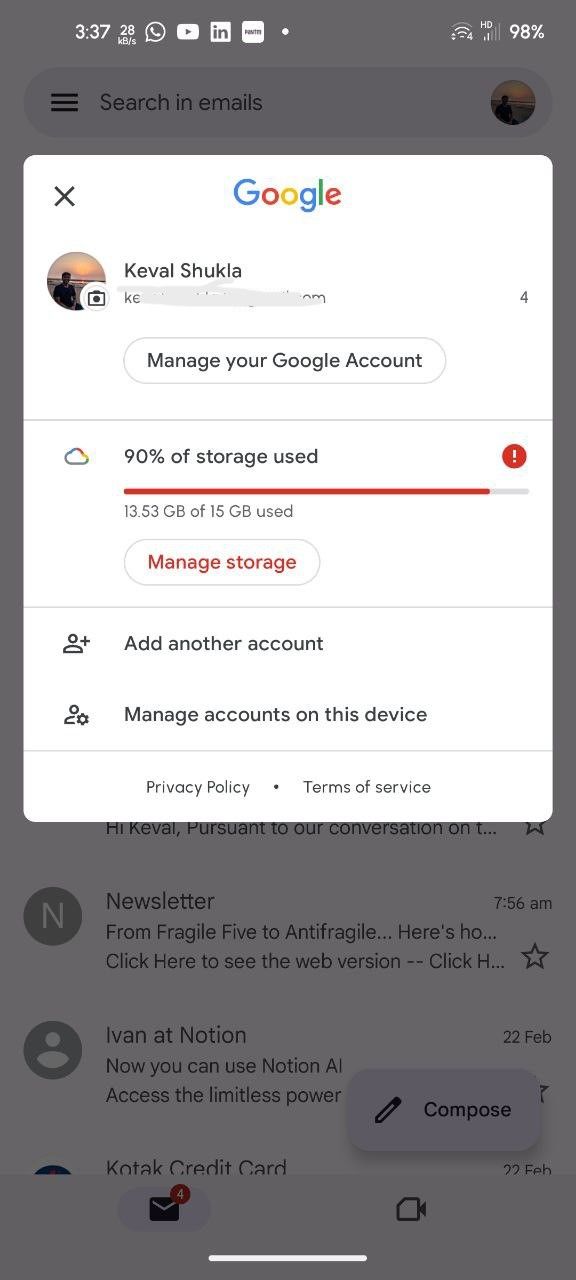In this screenshot of a phone screen, the time displayed in the top left corner is 3:37. Next to the time, there is an icon of a phone, an inbox symbol, and a signal strength indicator. On the far right, the battery level is shown to be at 98%. The screen is displaying a Google account page belonging to Kaveh Shukia, with a profile picture of Kaveh on a beach next to the name. Below the name, there is an option to manage the Google account. In a section further down, it states that 90% of the storage has been used, depicted by a nearly full red bar, indicating 13.53 gigabytes of the available 15 gigabytes have been utilized. There is an option in red text to "Manage storage" beneath this. Below that, there are options for adding another account and managing accounts on this device. The background of the screen is dimmed, but a couple of emails are visible, with one from a newsletter and another one from Ivan at Notion.